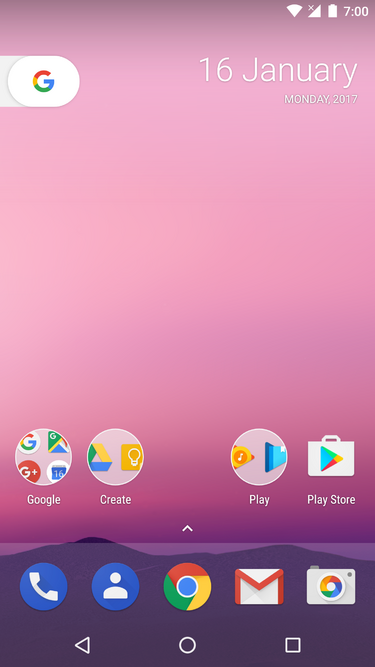This screenshot showcases a vibrant phone home screen with a visually striking background. The wallpaper features a gradient sky that transitions smoothly from pink at the top to purple near the horizon, accompanied by silhouettes of dark purple mountains at the bottom. On the upper right corner of the screen, the date "16 January" is prominently displayed, with the additional detail "Monday, 2017" positioned just below it. The top left corner features a sleek Google slide button with the iconic Google 'G' logo.

Toward the bottom of the screen are two rows of app icons. The top row consists of four apps: "Google," "Create," "Play," and "Play Store." The bottom row is slightly more populated with five apps: "Phone," "Contacts," "Chrome," "Gmail," and a "Photos" application. The organized layout and colorful background make this home screen both functional and aesthetically pleasing.